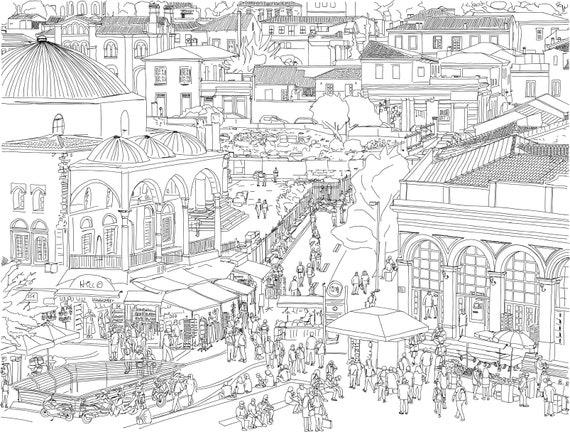This black-and-white pencil illustration depicts a bustling town square, reminiscent of a comic book with its finely detailed, thin lines. The scene is set in Monastiraki Square, Athens, Greece, showcasing a vibrant public space teeming with activity. On the left side of the illustration stands an architecturally distinct domed building with three smaller domes over a portico, evoking classical motifs. Adjacent to this structure, street vendors display a variety of clothes, tourist items, and other wares, attracting a diverse crowd of shoppers and visitors. 

In the bottom left corner, there is an enclosed corral-type structure, adding to the quaint charm of the scene. The right side features a prominent train station-like building with four arched openings, further hinting at the area's historic significance. Scattered throughout the square, numerous benches and kiosks serve as focal points for people to gather, relax, and socialize. The backdrop is lined with residential houses, adding depth and context to this lively urban tableau. Every element in the image—from the intricate architectural details to the animated crowd—is rendered meticulously in monochromatic tones, capturing the essence of a thriving, tourist-friendly cityscape.